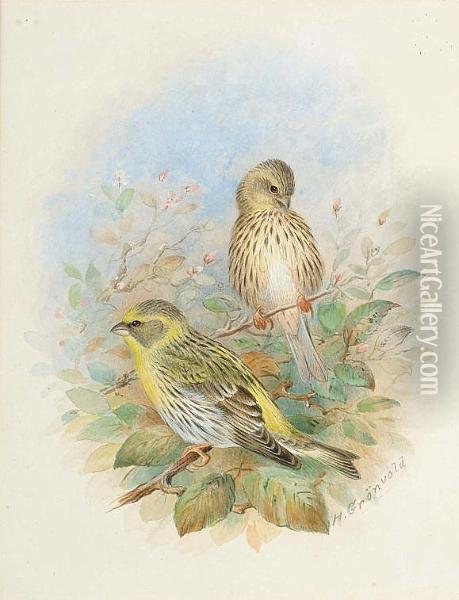This detailed pencil illustration showcases two birds perched on thin, leafy branches against a subtly faded blue sky. Positioned towards the right of the composition, vertical white lettering reads "NiceArtGallery.com," and in the bottom right corner, the artist's signature, "H. Gronvold," is visible. The lower bird, larger and facing away, features a vibrant yellow breast and tail, with white and brown feathers accented by black lines and patterns. Above it on a separate branch, a smaller bird gazes toward the viewer with a creamy white breast and tan feathers dappled with black. Both birds grip their twigs, surrounded by dark green leaves and light floral motifs, creating a serene and naturalistic scene.